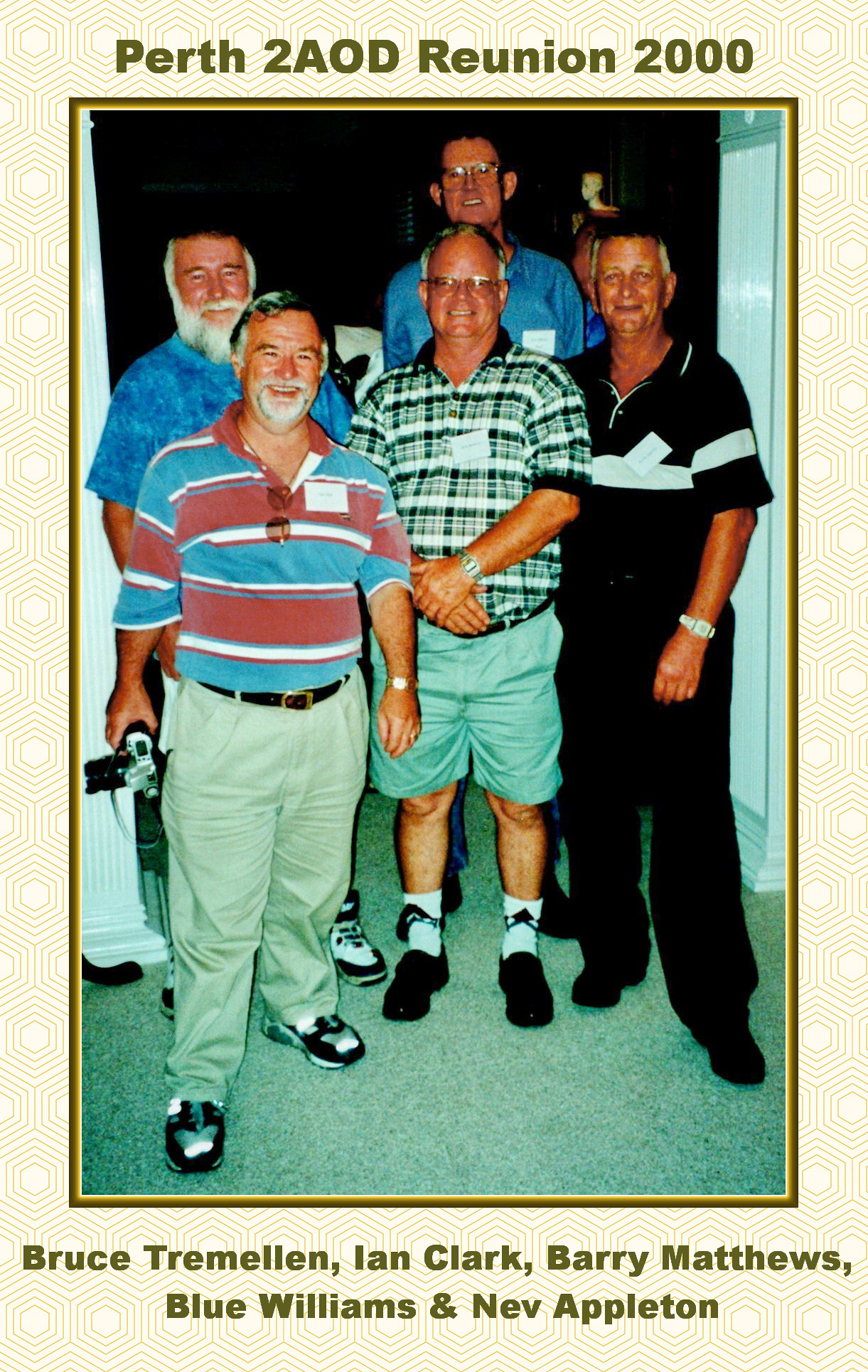The image showcases a reunion photo titled "Perth 2AOD Reunion 2000" with five men standing in two rows on a grayish-green carpet amid a black background. Text at the top reads "Perth 2AOD Reunion 2000," and at the bottom, in similar olive green text, are the names Bruce Tremelin, Ian Clark, Barry Matthews, Blue Williams, and Neve Appleton. The men, all smiling and older in age, are arranged with three in the front row and two taller individuals in the back row.

In the front row, from left to right:
- A man with a gray beard and short hair, dressed in a red, blue, and white striped polo shirt, khaki pants, and black and white sneakers.
- A bald man with glasses wearing a striped shirt in tones of green, black, and white, along with gray shorts, white socks, and black shoes.
- A clean-shaven man with gray hair, wearing a black polo shirt with a white horizontal stripe, black pants, and black shoes.

In the back row, from left to right:
- A man with a substantial white beard and mustache, sporting a blue shirt.
- A tall man with glasses and dark hair, also in a blue shirt.

The image is bordered with a black edge followed by an intricate yellow geometric pattern, creating a frame that ties together its nostalgic and celebratory theme.